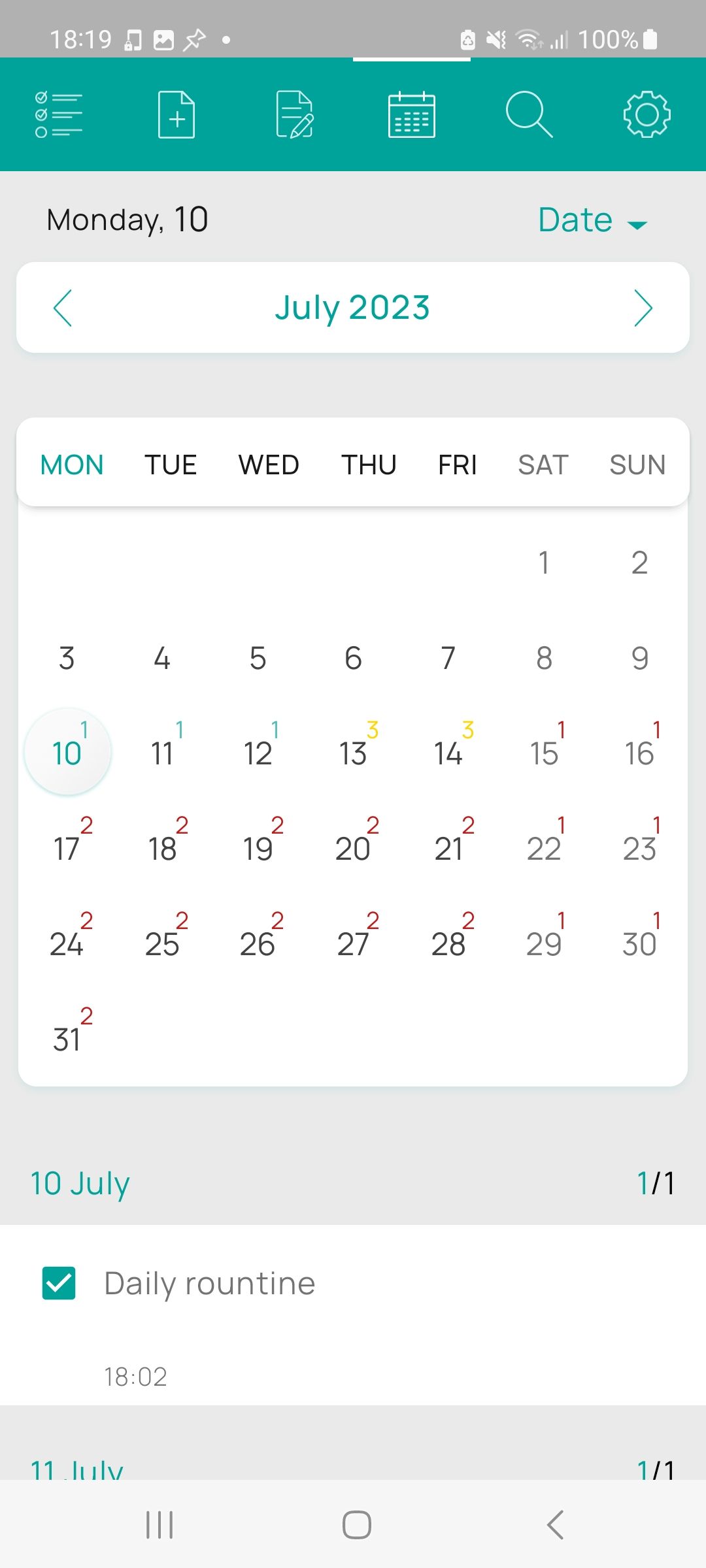On a website displaying a calendar, the current time is 18:19 with a fully charged battery at 100%. The date is set to Monday, 10th July 2023. Navigation arrows for the calendar are located to the right and left. The days of the week are labeled as MON, TUE, WD, THU, FRI, SAT, and SUN. Monday (MON) is highlighted in green, while the other days are in black. The month starts on Saturday the 1st and ends on Monday the 31st.

Details for July 10th include "10 July, 1 over 1" and a "daily routine" item with a checked checkbox beside it, timestamped at 18:02. Additionally, there are small numbers above certain dates: 10 (1), 11 (1), 12 (1), 13 (3), 14 (3), 15 (1), 16 (1), 17 (blank), 18 (blank), 19 (blank), 20 (blank), 21 (2), 22 (1), 23 (1), 24 (2), 25 (2), 26 (2), 27 (2), 28 (2), 29 (1), 30 (1), and 31 (2). The date "10" is also circled, indicating its selection or importance.